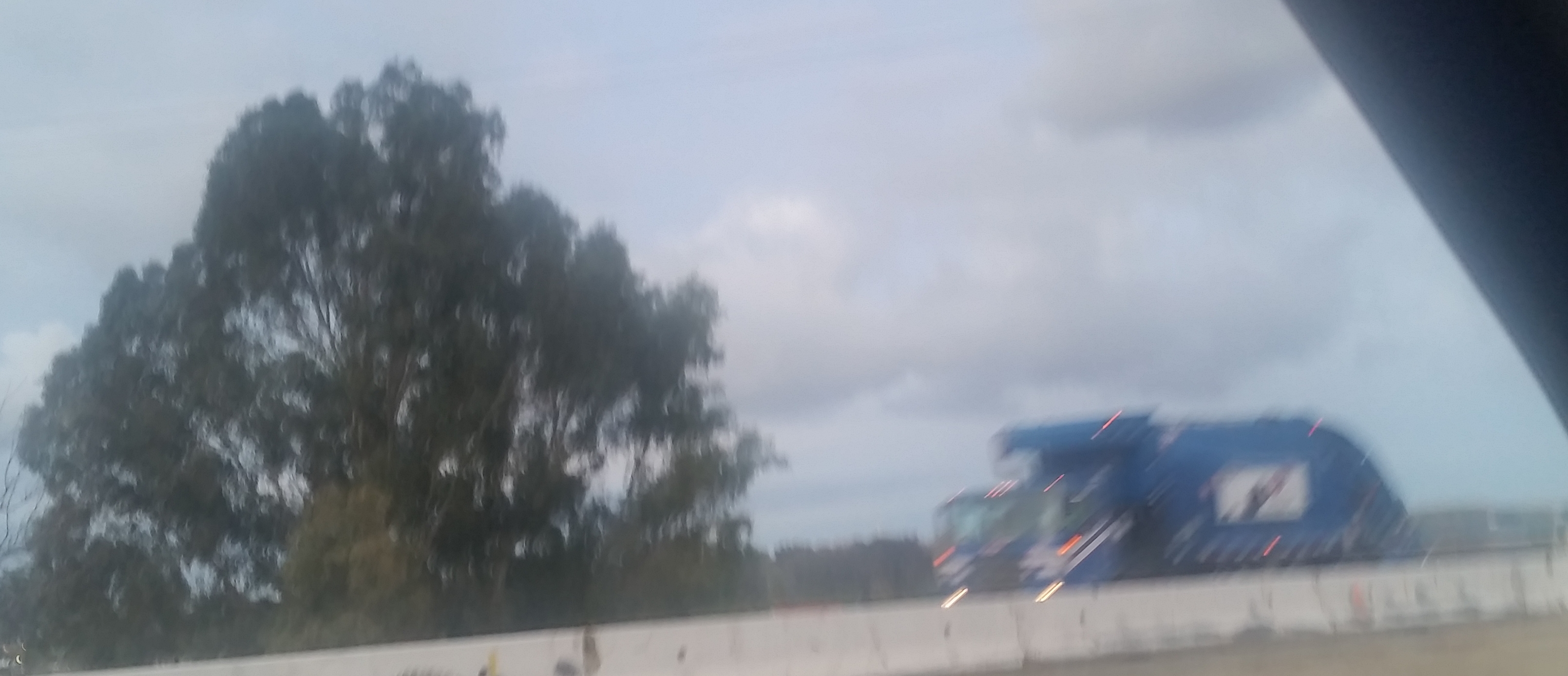This image, captured from within a moving vehicle, depicts a scene with a large green tree on the left and a blue garbage truck on the right. The tree dominates the left side of the frame, displaying plentiful dark green leaves and many branches. The blue garbage truck, which appears to be in motion, has a white square in the middle, a wide front bumper, and some orange elements including lights. The background shows a blend of white and gray clouds with some patches of blue sky visible near the tree. A concrete barrier, like those found on highways, runs horizontally across the lower part of the frame, separating the viewer from the moving truck. The overall image is very blurry, emphasizing the motion and suggesting it was taken from a traveling vehicle. In the upper right corner, there is a black area that could be part of the vehicle from which the photo was taken.